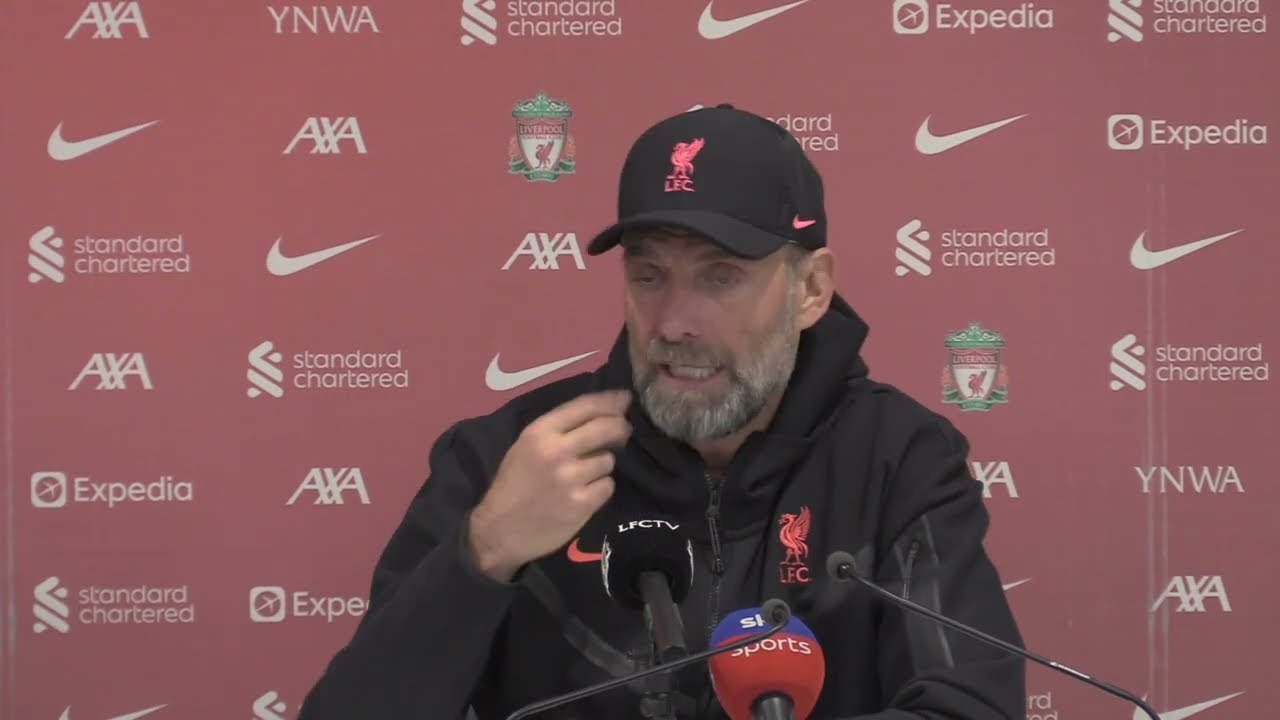The image captures a sports figure, likely a coach, seated at a press conference. He is wearing a black jacket with a red "LFC" logo on one side of his chest and a red Nike swoosh on the other. His black cap also features the same red "LFC" logo and a red Nike swoosh. Sporting a gray beard and mustache, he appears to be in mid-speech. In front of him are multiple microphones, including a prominent one from Sky Sports and another labeled "LFC TV." The backdrop behind him is a light red or pinkish hue, adorned with white Nike swooshes and various sponsor logos such as AXA, Expedia, and Standard Chartered, which repeat in different configurations. Additionally, a distinctive red and green shield-like emblem featuring a bird is present both on the backdrop and on his attire, suggesting its significance to the team or organization he represents.